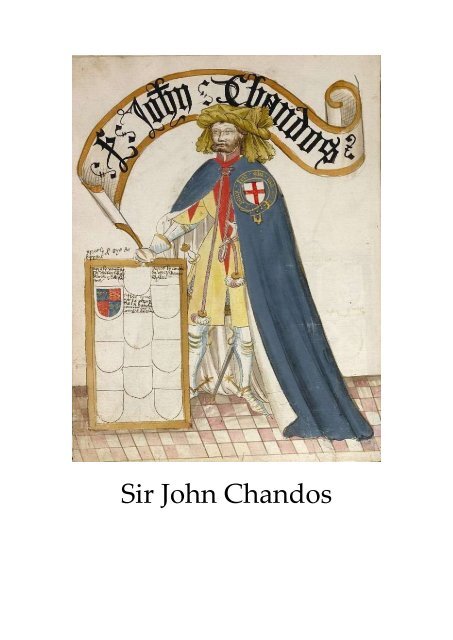This detailed illustration depicts a medieval lord named Sir John Chandos, as identified by the gothic script text below the image, with a modern print spelling C-H-A-N-D-O-S. The distinguished figure stands confidently at a podium, which he appears to be holding. Sir John is adorned in a striking long blue cape over red and yellow robes. His attire is complemented by white tights and shoes. The blue cloak features a crest on the shoulder with a white background and a red cross in the center. He wears a yellowish light brown head wrap, possibly a turban, and has a matching yellow beard. 

Above his head, a wavy scroll inscribed with "John Chandos" in Latin adds an additional layer of grandeur to the illustration. Next to him is a sign with various painted shields, contributing to the heraldic theme of the artwork. The composition provides a robust visual tribute to the historical figure set within the medieval era.